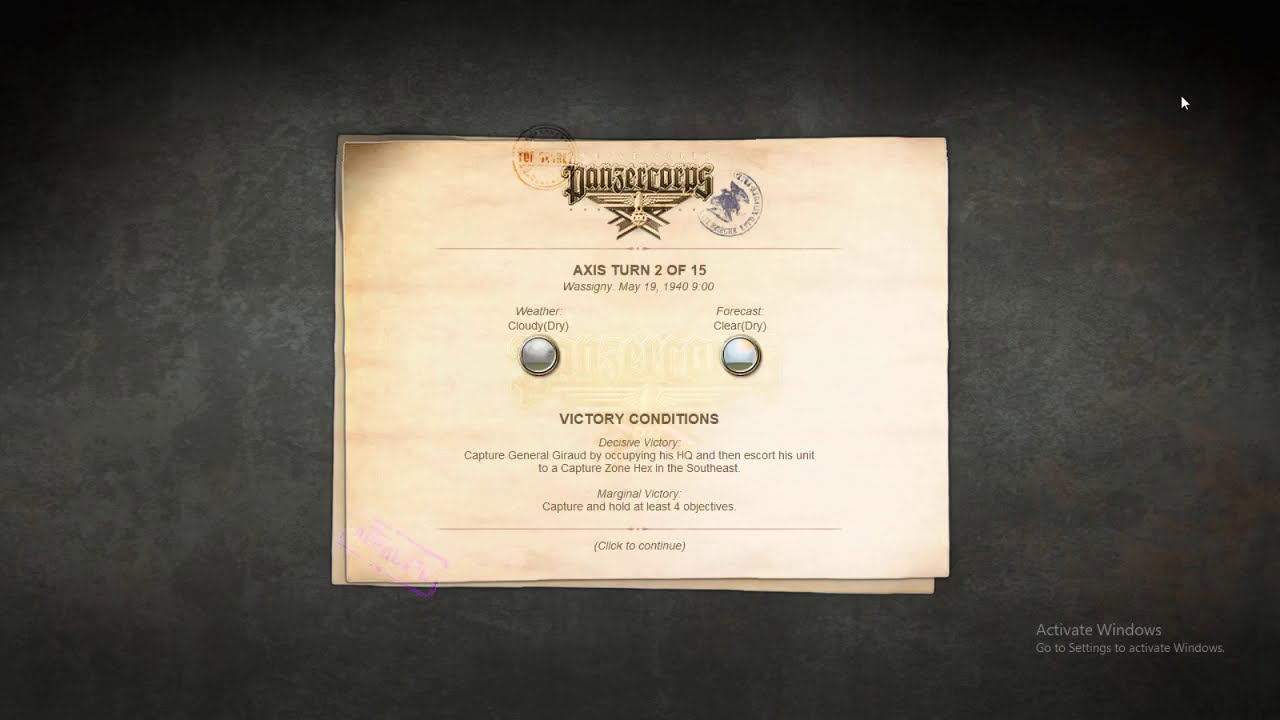The image displays a screenshot from a video game, framed by a dark charcoal or gray background that transitions to a lighter gray toward the center, with a black border around the edges. At the bottom right corner, there's a faded message reading "Activate Windows. Go to settings to activate Windows." The main focus is a certificate-like document resembling parchment paper, positioned centrally, with a decorative shield at the top, reminiscent of a Medal of Honor. The document is marked with two stamps: a blue one and a partially visible red one, with the latter bleeding onto the background. Text on the certificate includes: "Axis turn 2 of 15," "Wassonie, May 19th, 1940, 9 o'clock," "Weather: cloudy, dry," and "Forecast: clear, dry." Detailed victory conditions are outlined, specifying objectives such as capturing General Girard by occupying his HQ and escorting him to a capture zone in the southeast for a decisive victory, or capturing and holding at least four objectives for a marginal victory. The image is a horizontally-oriented rectangle, with the objective screen appearing as a central square, punctuated by a black and gray border.